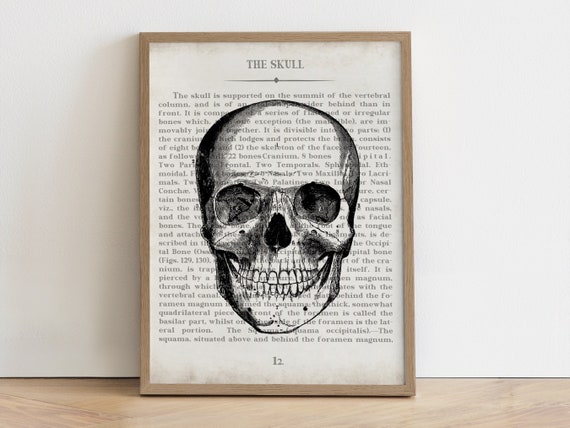The image depicts a framed page from a book, titled "The Skull," resting against a white wall with either a hardwood floor or a light brown table beneath it. The frame is made of light or tan wood. The page inside the frame features a black-and-white line drawing of a human skull with prominent details such as empty eye sockets, a visible nose cavity, and a full set of teeth. The drawing is superimposed on text that begins with the words, "The Skull is supported on the summit of the vertebral column," and continues down the page. A line separates the title from the rest of the paragraph, making the overlaying text difficult to read through the skull illustration. Additionally, there are two lines with a diamond shape in the middle, situated beneath the title and above the primary text block. The setup resembles an artistic portrayal of anatomical literature.